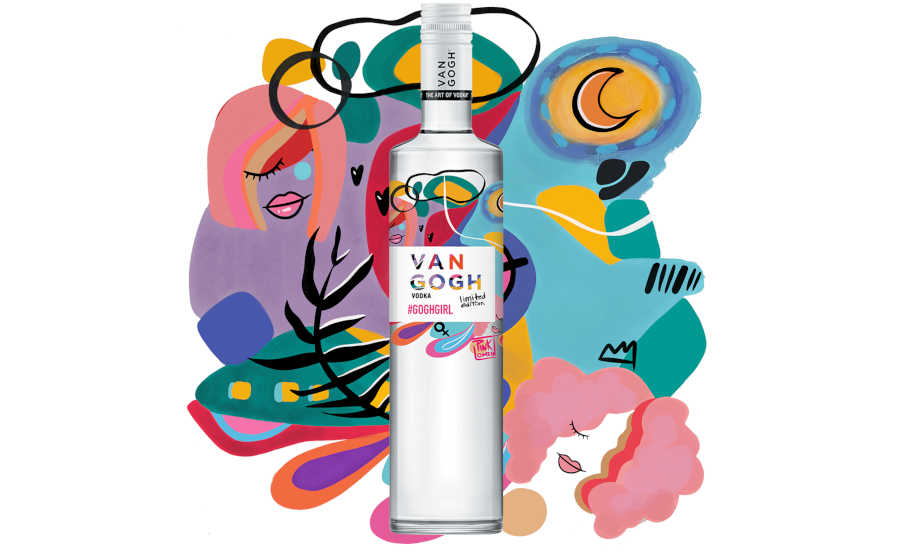In the image, we see a silver-colored bottle of Van Gogh Vodka with a white screw-top cap and two black horizontal bands around the upper neck, one of which appears to have a black lanyard or lace attached. The label in the upper center of the bottle prominently features the words "Van Gogh Vodka" with additional smaller black text beneath it, including hashtags and the term "limited edition." Below the label, there's a depiction of the female biological sign. 

The design on the bottle is vibrant and abstract, featuring a mix of pink, purple, teal green, and bright blue colors. The artwork includes various elements such as a woman’s face with distinctive pink hair and lips, another eye and lips in the lower right, and a crown above her head. This artistic style extends into the background, which mirrors the bottle's artwork, suggesting a tropical scene with elements like plants, a moonrise, and an ocean, all artistically intertwined. The background likely includes a larger rendition of the same abstract imagery seen on the bottle, emphasizing a vivid and eclectic theme suitable for a marketing advertisement.